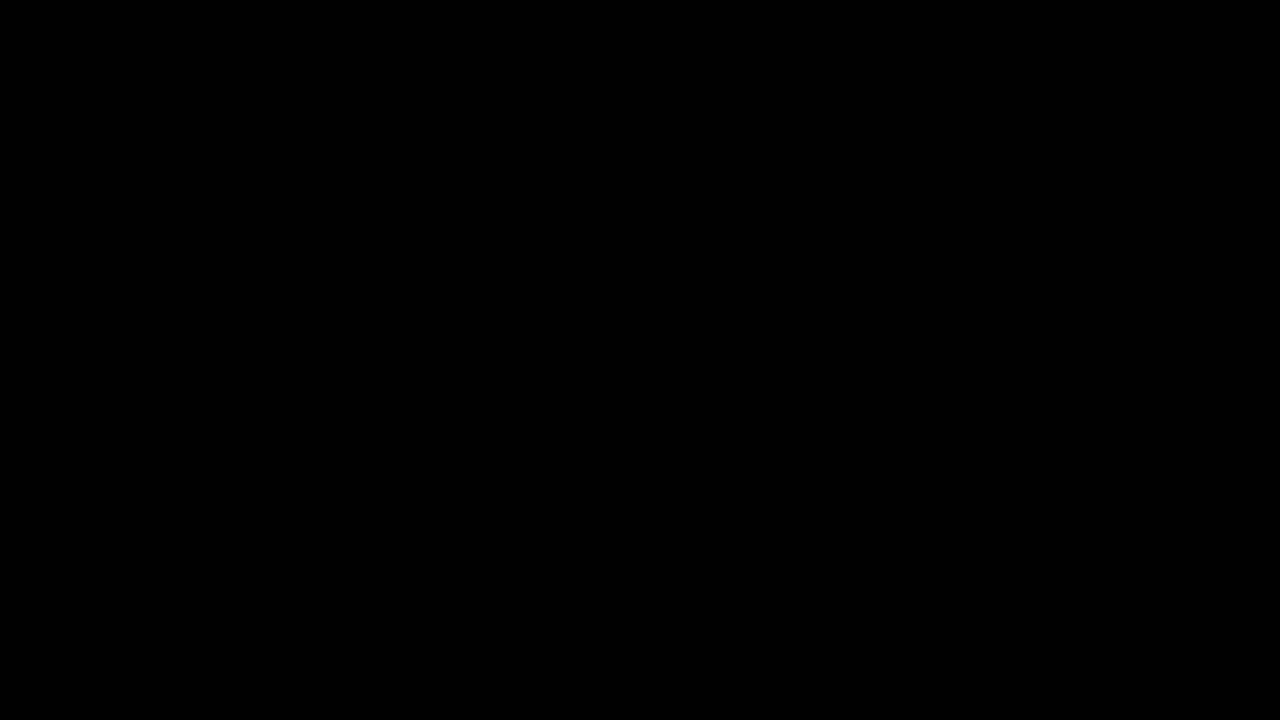The image depicts a completely black rectangle, void of any detail or visible elements. The dark expanse is uninterrupted and uniform, suggesting no errors or loading issues—it is simply an entirely black and blank screen. The dimensions of the black rectangle appear to be nearly twice as wide as it is high. Despite the potential for a glitch, there is no indication of error, merely an intentionally pitch-black image filling the frame from edge to edge.